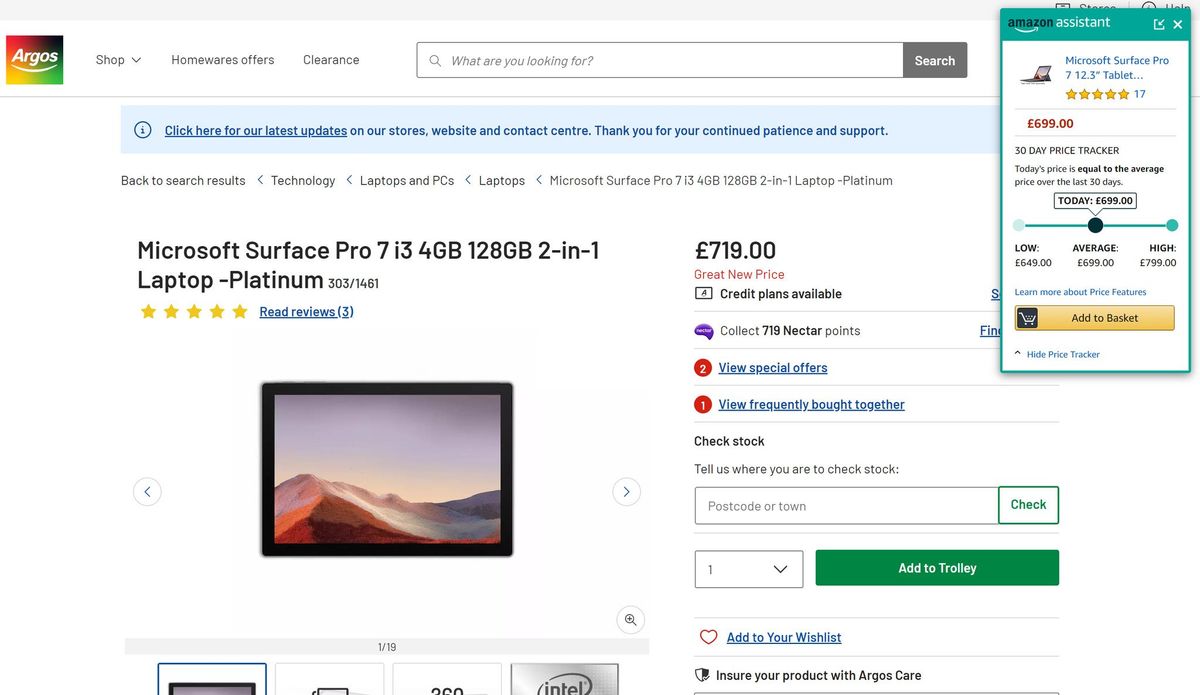The image is a detailed screenshot from a website that resembles Amazon but is more likely a sub-site or an affiliated platform. At the top, there is a thin gray bar with text on the right side, partially obscured by a pop-up window. Below this, the header prominently displays the Argos logo, indicating that the site relates to Argos, a popular UK retailer known for its electronics and homewares.

The navigation bar below the logo features buttons for "Shop," "Homewares," "Offers," and "Clearance," all in gray. To the right of these buttons, there is a white search box labeled "Search." Beneath the navigation bar, a blue banner with blue text, underlined for emphasis, reads "Click here for our latest updates," followed by information about store updates, website updates, and contact center details, thanking customers for their patience and support.

The main content below this features product information for a "Microsoft Surface Pro 7." The product is described as having an Intel Core i7 processor, 4GB of RAM, and 128GB of storage, priced at £719. A pop-up from the Amazon Assistant suggests that the same product is available elsewhere for £699, noting a £20 savings. Instead of using the term "cart," the site uses "trolley" for adding items, reflecting the UK terminology.

On the bottom left, there are partially visible images showing different angles of the Microsoft Surface Pro 7, enhancing the product display section.